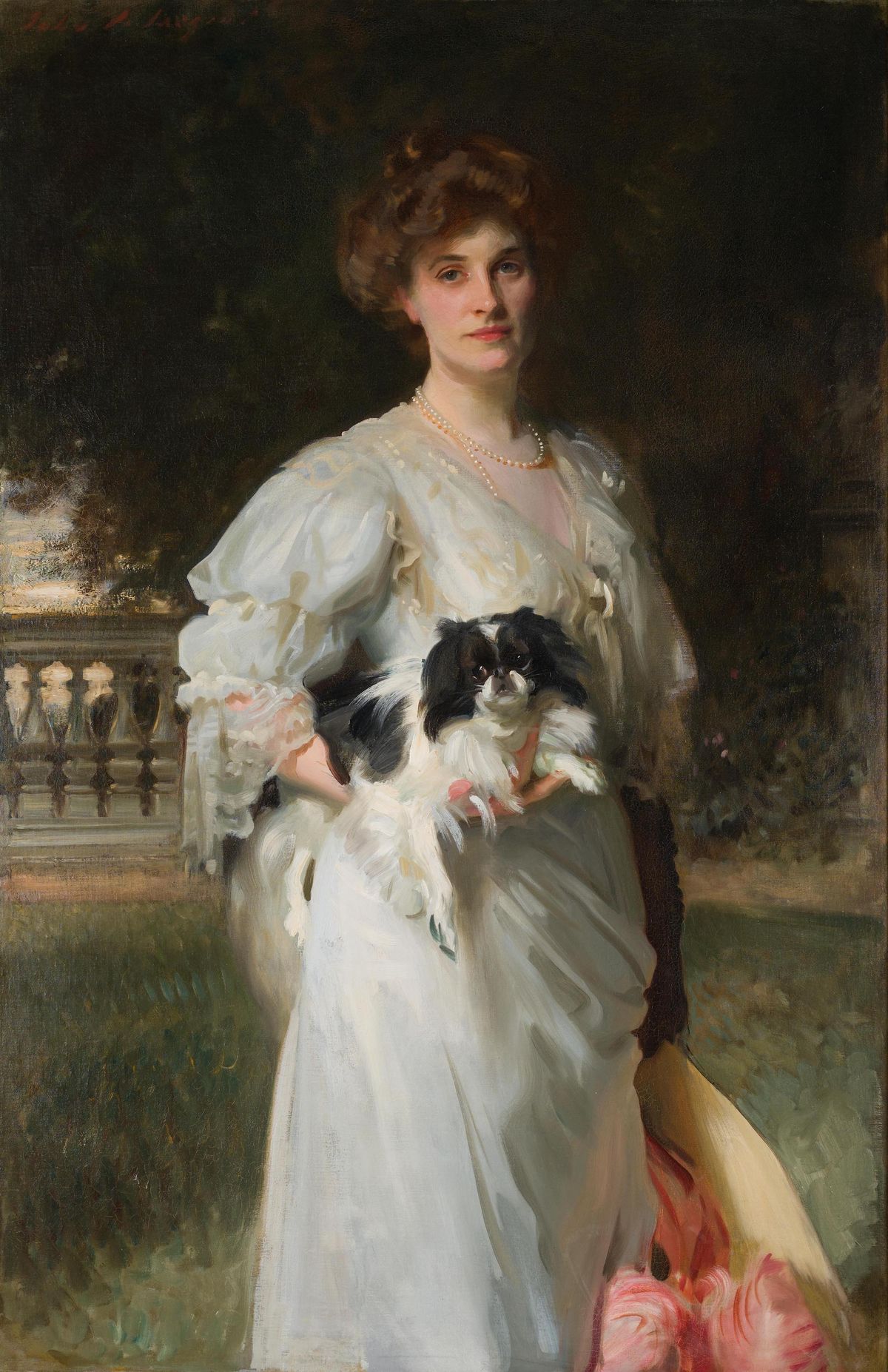The image depicts an old, historically-styled painting of a youngish woman, likely in her late 20s or early 30s, who appears to be part of the aristocracy. She stands gracefully in the middle of a garden courtyard against the backdrop of a large tree and a stone balcony or fence to her left. The woman has curly brown hair and is wearing a flowing white lacy dress, reminiscent of a wedding gown, adorned with a pearl necklace. In her left hand, she carries a bouquet of flowers, while her right arm cradles a small black and white dog, possibly a Pomeranian, featuring a black face with long fur around its ears and black patches on its body. The overall scene suggests a serene, elegant outdoor setting typical of classical portraiture.